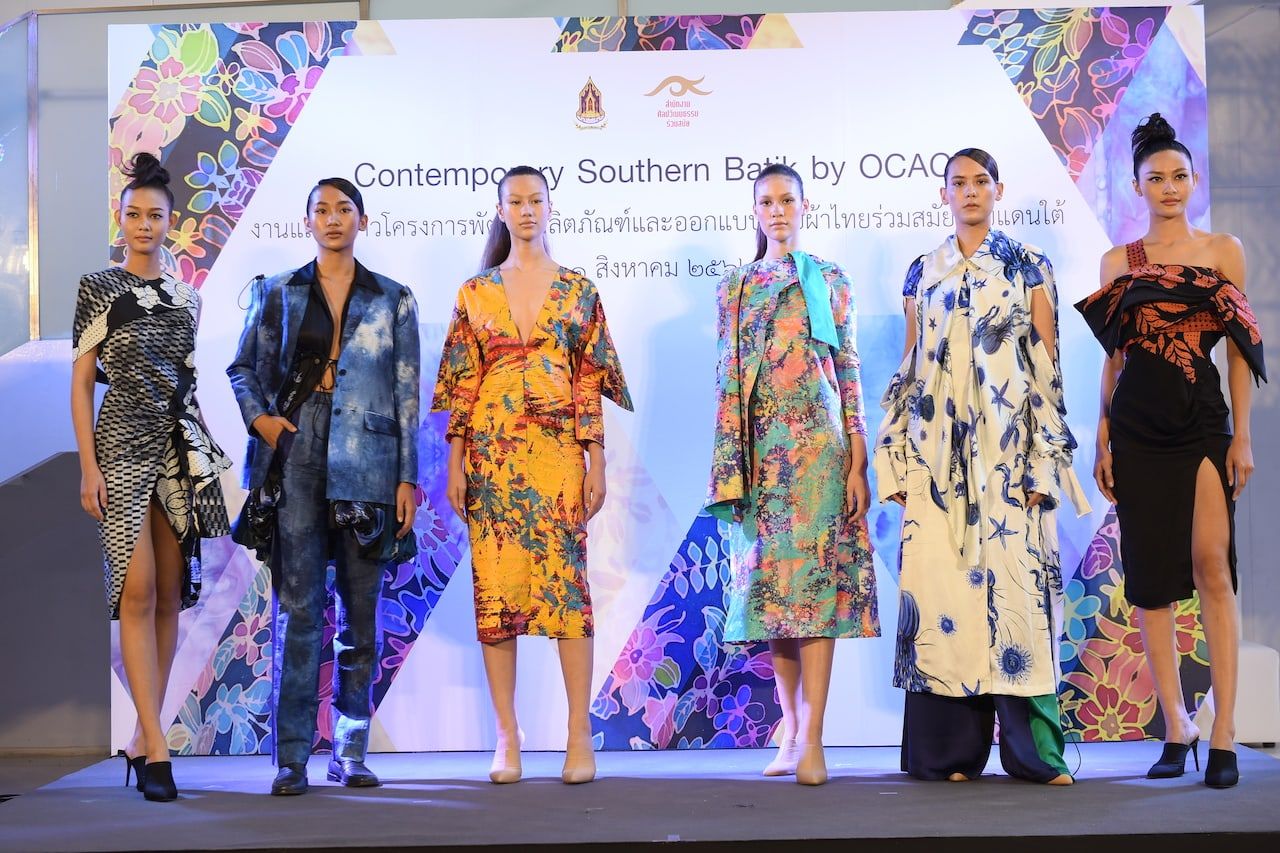In this image, six young Thai women are standing in a row, participating in what appears to be a fashion show or dress demonstration. They are positioned in front of a backdrop which reads "Contemporary Southern Batik," flanked by additional text in a Cyrillic or Thai script.

Starting from the left, the first woman is wearing an eye-catching black and white print dress, adorned with a matching scarf draped over her left shoulder and extending to her right arm. Her dress is notably slit at the middle, revealing her upper thighs, and she complements the look with black high-heeled shoes.

The second woman sports a stylish ensemble consisting of a blue and black print jacket and dark pants, complete with a satchel slung over her right side. Her look is finished off with short hair and black shoes.

The third woman dons a vibrant white, red, yellow, and blue print dress that reaches just below her knees, adding a touch of floral elegance to the lineup. 

Next, the fourth woman chose a conservative yet colorful dress with shades of light blue, yellow, purple, and red. She accessorizes with a light blue shawl over her left shoulder, and a matching scarf that extends from her right shoulder to below her wrist, with the dress itself ending below her knees.

The fifth woman is showcasing a blue and white floral print jacket with exposed forearms, paired with what appears to be purple pants peeking out beneath the jacket. She adds a touch of whimsy with a mostly white dress featuring blue sea life prints.

Finally, the sixth woman stands out with a stylish black and orange dress with a pattern resembling upside-down leaves. The dress features a bare left shoulder and a single strap on her right shoulder, complemented by a dramatic thigh-high slit on her left side. She completes her attire with black shoes.

The women are all positioned on a gray stage, adding a uniform backdrop to their varied fashion statements.